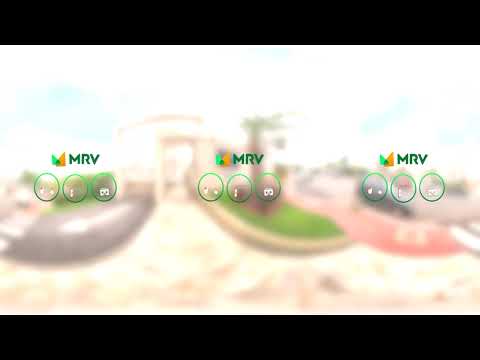The image depicts a scene viewed through a frosty, blurred filter, rendering everything indistinct. Dominating the foreground are three identical logos, each featuring overlapping orange and green triangles with the initials "MRV" prominently displayed beneath the triangles in green capital letters. Below each set of initials, three green circles are arranged in a line gradient, from light green at the top to dark green at the bottom. Inside these circles are faint white icons—the first circle contains two white figures, the second houses a cylindrical shape, and the third has a shape resembling either a face or a game controller. The logos repeat vertically across the image. In the hazy background, against bright white light, there's a vague outline of a road or entrance, surrounded by what seem to be green grass and possibly a building or palm trees. The top and bottom of the image feature black bars, further adding to the indistinct, frosted-glass effect.